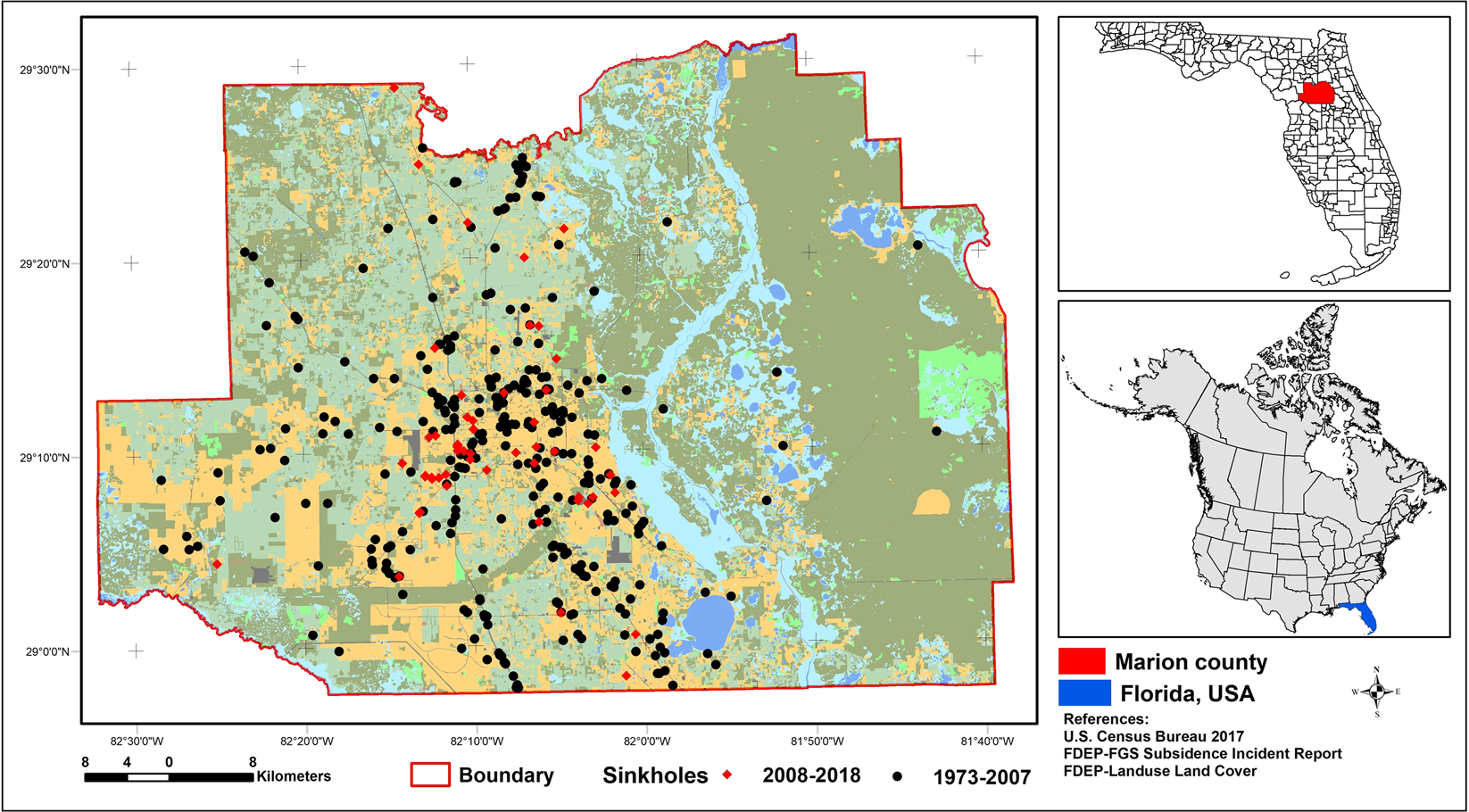This detailed visual representation is of Marion County, Florida, USA, featuring data from multiple sources including the U.S. Census Bureau's 2017 report and the FDEP-FGS Subsidence Incident Report, focused primarily on documenting sinkholes. The central map on the left pane, encased within a red border, displays Marion County with extensive details including geographic coordinates and a color-coded key. A red boundary outlines the county, while red circles indicate sinkholes identified between 2008 and 2018, and black dots represent those from 1973 to 2007. The distribution shows a greater number of older sinkholes compared to more recent ones. Dark and light green patches denote different land cover types, with numerous water bodies visible throughout. 

Inset to the right, the top image shows a monochromatic map of Florida, highlighting Marion County in red. Below it, another graphic of the North American continent, minus Mexico, depicts Florida in blue for context. This portion of the image provides orientation, showcasing Marion County's location within the broader state and country. Additional elements in this imagery include a compass for direction, a scale bar in kilometers, multiple legends, and textual references to the data sources and land use. The overall composition is meticulously detailed, illustrating not just the location but also the prevalence and timeline of sinkholes within Marion County over several decades.